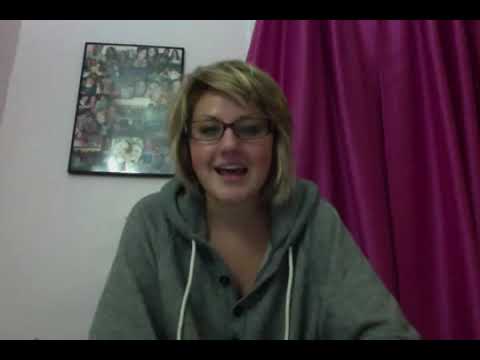This image appears to be a screenshot of a woman engaged in a video chat, as suggested by the slightly blurry quality and the horizontal bars at the top and bottom of the frame. The woman has a Caucasian skin tone and is captured from the chest up. She is wearing a gray button-up hoodie with white pull strings and dark brown oval-shaped glasses. Her shaggy, chin-length blonde hair features slight bangs. The woman is smiling slightly while speaking, with her mouth open. In the background, there is a vibrant, deep violet-red curtain on the right side of the image and a framed photo collage on the off-white wall to the left, though the collage appears somewhat blurry and partially obscured by a glare on the glass.